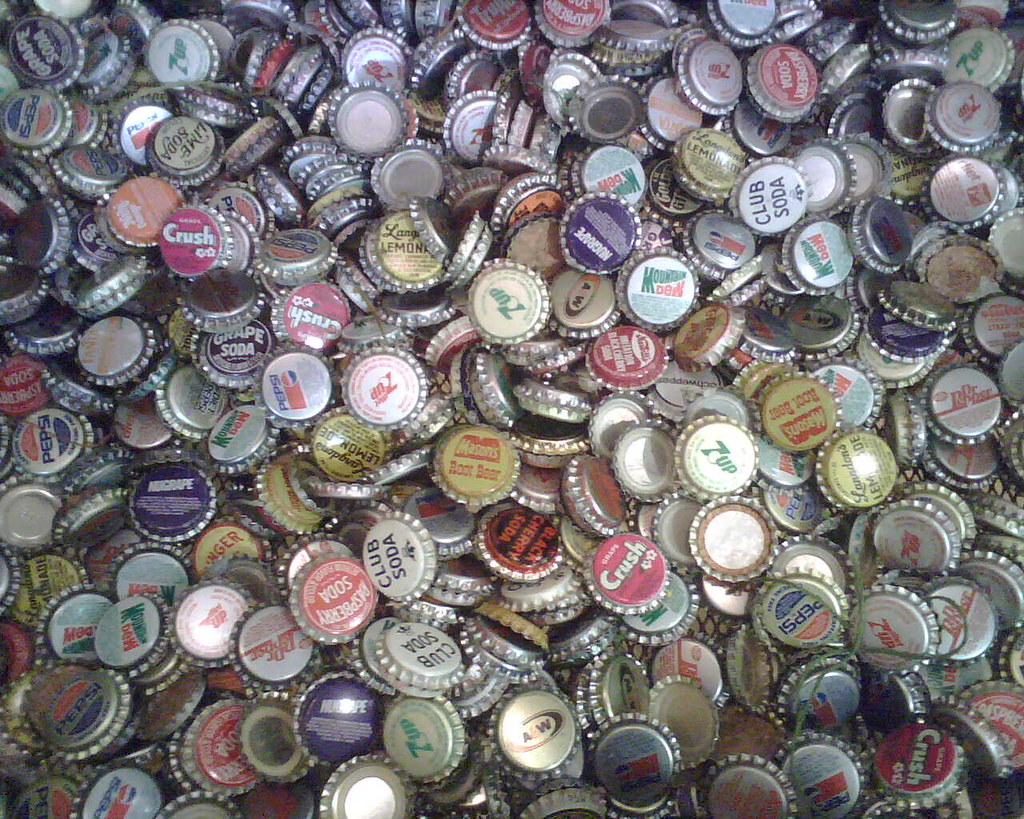The image is a densely packed collection of various bottle caps, creating a vibrant and chaotic scene. Among the multitude, familiar brands stand out: Mountain Dew caps with their green and red logo, Club Soda caps, Crush caps in red, A&W caps in orange and black, Pepsi caps with their distinctive logo, and 7UP caps with their green logo. Additional caps include Lime Soda, Black Cherry Soda, and Grape Soda in various color combinations. The caps are stacked on top of each other, filling the image with a myriad of colors and designs, each with a distinct circular shape and branded center.